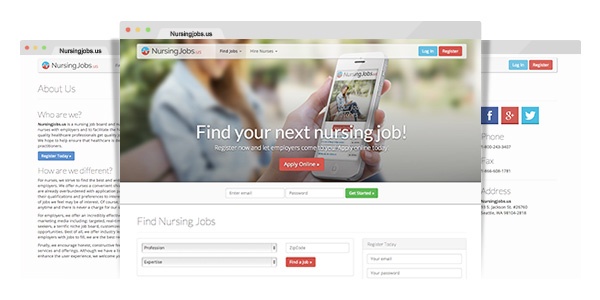The image displays a webpage with a clean, white background. Dominating the center of the screen is a pop-up window featuring a large photograph of a woman with long hair, dressed in a light blue shirt. Positioned in front of her is a hand holding a smartphone, with the text "Find your next nursing job" inscribed in white across both the shirt and the smartphone.

To the left of the pop-up, there is some introductory or explanatory text written in black, directly on the white background of the webpage. To the right of the pop-up, three social media icons are neatly aligned: a white 'F' on a blue square representing Facebook, a 'G' with red accents symbolizing Google, and a white bird on a blue square indicating Twitter.